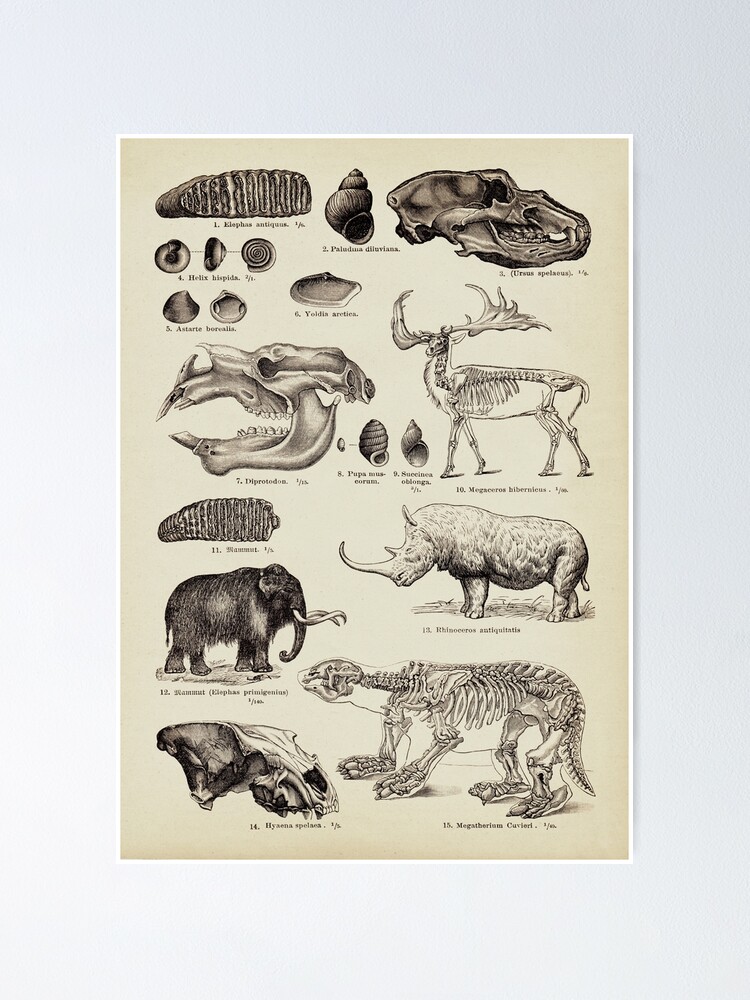This detailed scientific diagram depicts various prehistoric animals and fossils, meticulously rendered in black and white shading on a cream-colored background with a small white border. Prominently featured is a woolly mammoth, distinguishable by its two long tusks and trunk. Another notable figure is a large moose-like skeleton with expansive antlers. A sketch of an ancient rhinoceros showcases a prominent long front tusk. Additionally, the diagram includes several shells, including a small snail, and multiple intricate fossil renderings. A saber-toothed tiger skeleton, marked by its distinctive elongated teeth, is also present. Various skulls, including one with prominent tusks resembling a squirrel's, are dispersed throughout. Despite the tiny, unreadable text, the scientific precision of the pencil or pen sketches is evident, suggesting it as an educational tool likely displayed in a classroom or college setting.